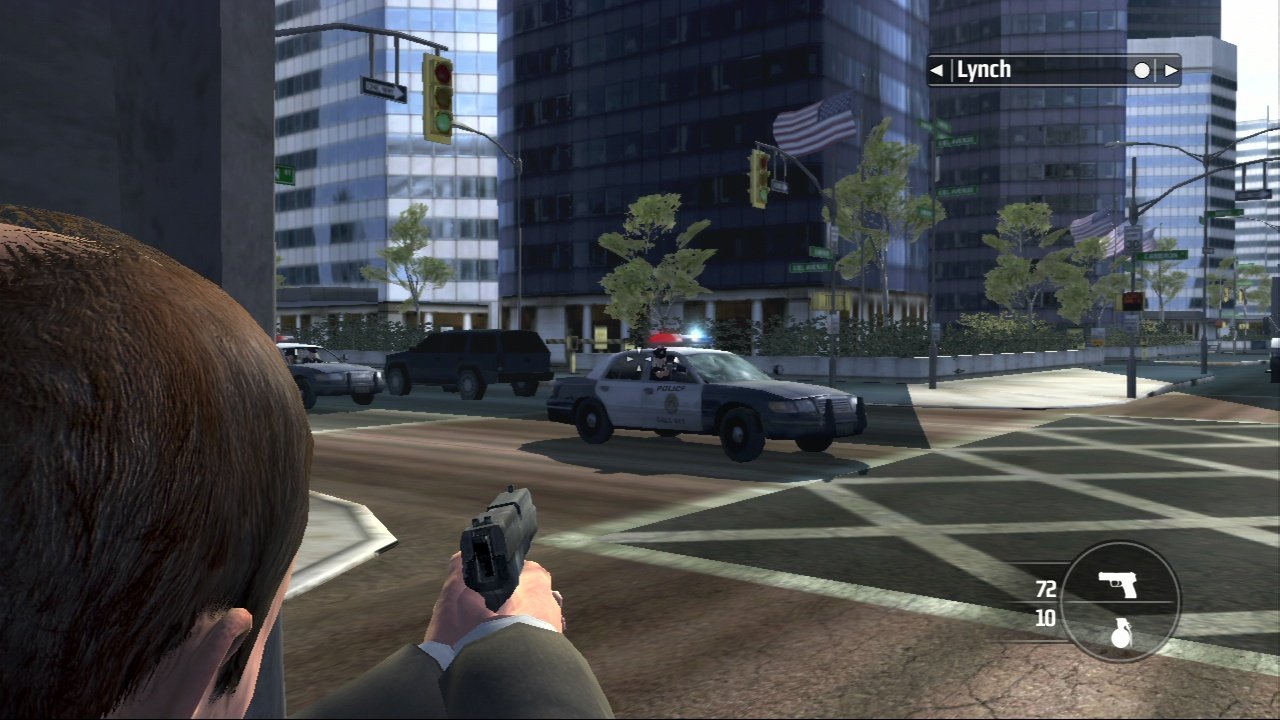In this detailed screenshot from a video game, a tense urban scene unfolds in what appears to be a large city, possibly modeled after New York City, characterized by its towering skyscrapers and bustling atmosphere. At the center of the action is a man with brown hair, dressed in a sharp gray suit. He stands with a determined expression, wielding two handguns, one in each hand, both aimed menacingly at an approaching police car. The police vehicle, with its emergency lights flashing urgently, is in the process of turning right into a busy intersection. The dramatic lighting and realistic cityscape enhance the intensity of the moment, capturing the high-stakes confrontation in vivid detail.